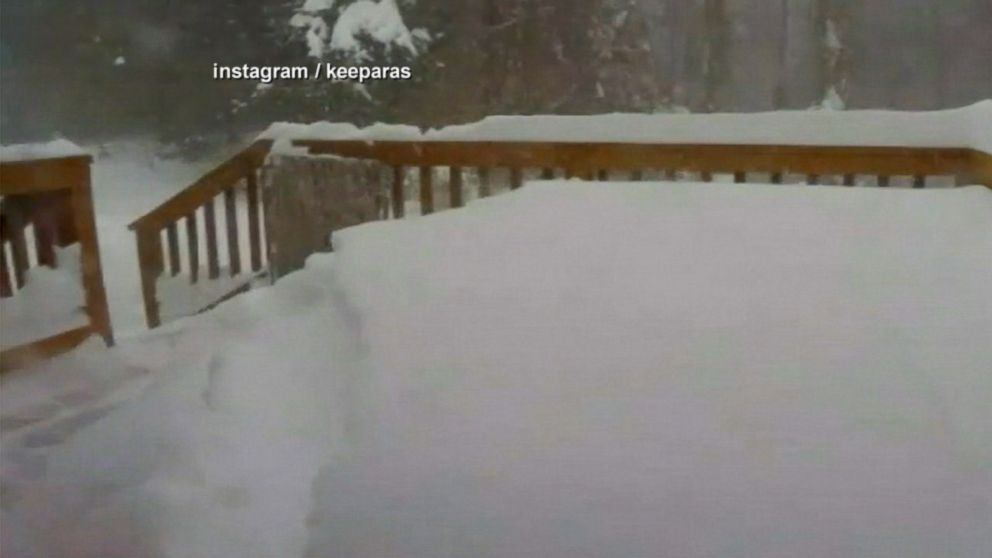This photograph captures a heavily snow-covered, wooden deck with light brown angular rails nearly buried under an estimated four feet of snow. The depth of the snow reaches almost to the top of the three-foot railing, leaving only the outer edges visible. A set of stairs adjacent to the deck appears partially collapsed under the weight of the snow. In the background, blurred woods with bare trees surround the scene, except for a lone cedar tree, which is also laden with snow. The text overlay reads "Instagram / Kiporos," suggesting the image was shared on that platform. The overall setting evokes a tranquil winter atmosphere, possibly indicative of a cabin or ski resort location.